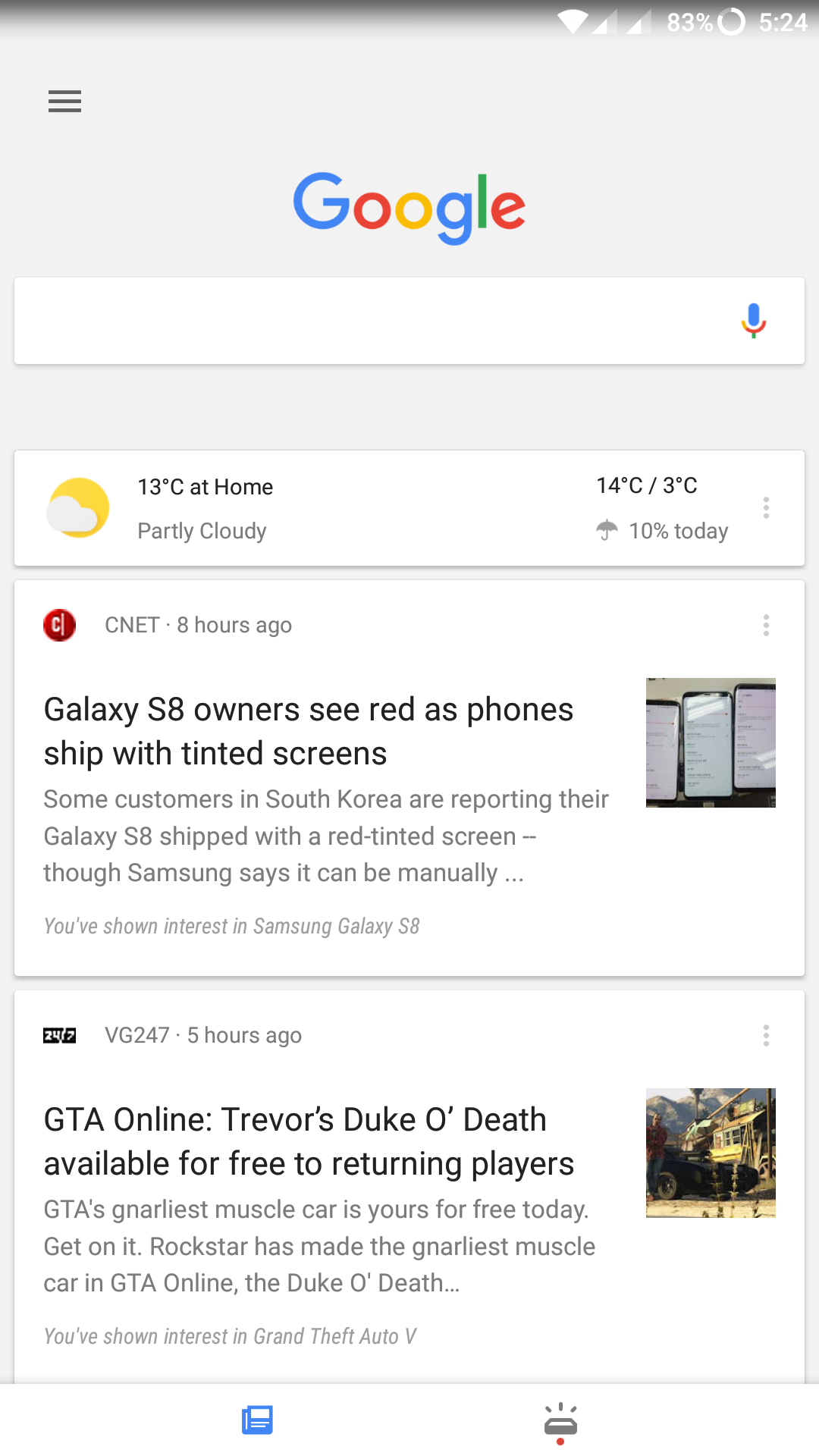This image is a screenshot of an Android phone, easily identified by the status bar icons in the top right corner. The screenshot showcases the Google homepage. At the top of the screen is the iconic Google search bar, crowned by the Google logo. Below the search bar, there is a weather update indicating it is 13 degrees Celsius and partly cloudy at the user's home. Additional weather details show a high of 14 degrees Celsius and a low of 3 degrees Celsius, with a 10% chance of rain as depicted by an umbrella icon.

Beneath the weather information, the screen displays tailored content. The first article is from CNET, titled "Galaxy S8 owners see red as phones ship with tinted screens." The article notes that some customers in South Korea have reported receiving Galaxy S8 phones with red-tinted screens, although Samsung claims this can be manually adjusted. 

The second article, from VG247, was posted five hours ago and announces that "GTA Online: Trevor's Duke O'Death is available for free to returning players." It details that this highly popular muscle car in GTA Online can now be obtained for free, catering to users interested in GTA 5. The Google homepage presents these articles because the user has previously shown interest in the Samsung Galaxy S8 and GTA 5, respectively.